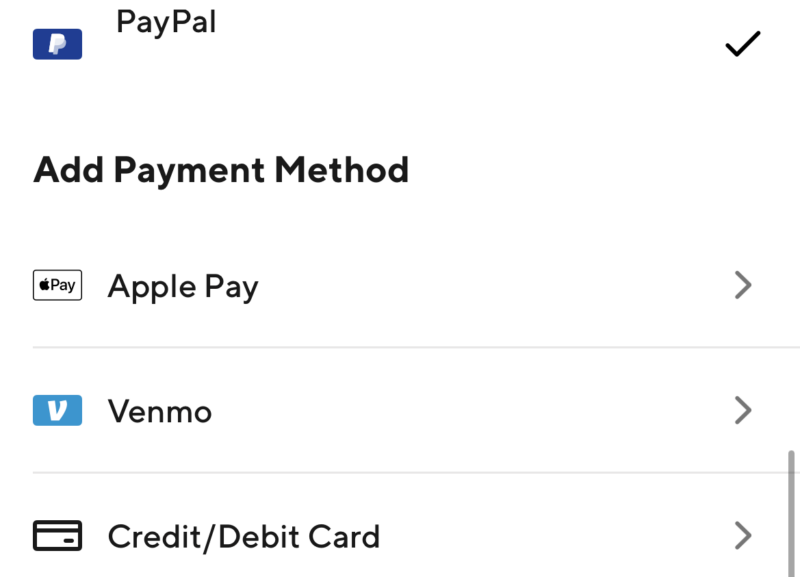The image displays a PayPal payment method screen against a white background, occupying the entire space. In the upper left corner, "PayPal" is prominently displayed alongside the PayPal logo. Below this, a list of payment methods is presented in a vertical row. The topmost option is "PayPal," marked with a prominent checkmark to its right, indicating it as the selected method. Beneath it, the text "Add Payment Method" appears without bold formatting.

The list continues with three additional payment options: "Apple Pay," "Venmo," and "Credit/Debit Card." Each of these options has a right-facing arrow next to it, suggesting further actions or additional details can be accessed. Gray lines separate each payment method from the next, maintaining a clear visual structure.

On the right side of the screen, from the bottom right corner and extending slightly upwards just past the Venmo option, another gray line is visible. The overall color scheme includes black, white, gray, blue, and turquoise, contributing to a clean and uncluttered appearance.